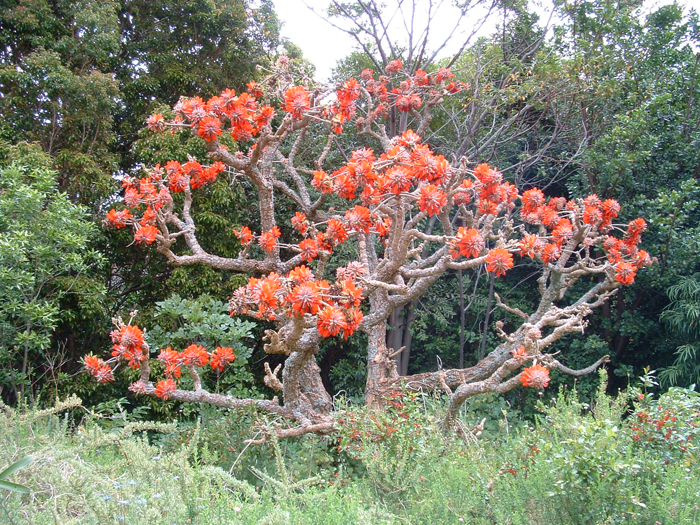This horizontal rectangular photograph captures a vibrant scene centered on a large, bush-like plant without leaves, showcasing its thick, grayish-brown trunks and spiky branches. The plant, which occupies a prominent space in the middle of the image, is adorned with bunches of peachy-orange flowers at the ends of the branches, possibly indicating a subtropical species. The ground around the bush is covered in light green weeds and various shorter vegetation, creating an untamed, natural feel. The background is filled with taller green trees that stretch up to the top of the image, leaving a small break in the center where the grayish-blue sky is visible without any distinct clouds. This setting, with its lush vegetation and flowering centerpiece, evokes a serene summer day immersed in the heart of nature.